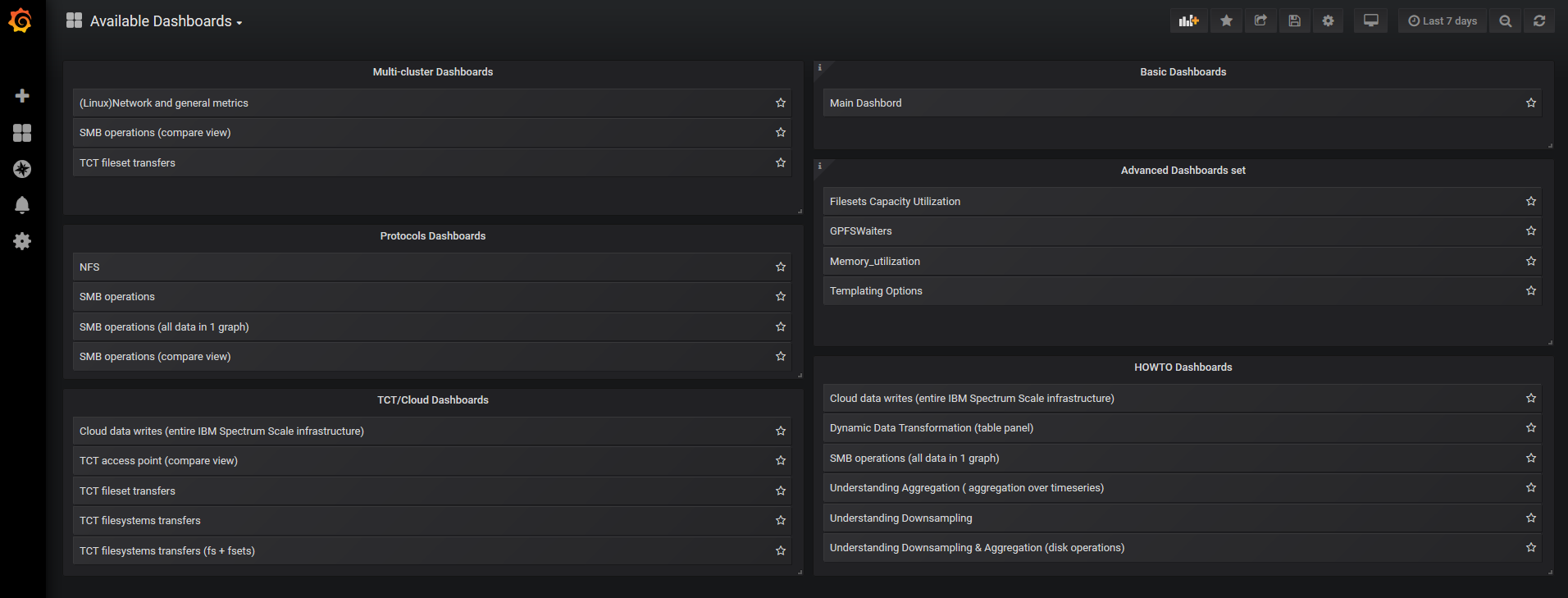The image depicts a screenshot of a computer dashboard interface, likely from a desktop or laptop computer. In the top left corner, there is a distinctive orange and yellow swirl design. To the right of this design are four light gray squares labeled "Available Dashboards," accompanied by a drop-down menu for options. The left panel features a plus sign, a repeat of the four gray squares, a circle icon, a notification bell, and a settings gear icon.

On the top right-hand side, there is a star icon for favorites and a floppy disk icon for saving. Additionally, there is a comment section and a search bar set to filter results from the last seven days. A circular arrow refresh icon and two navigation arrows are also present.

The main interface displays two side-by-side stacks of categories against a black background with small, white text, which is challenging to read due to its size. The overall layout suggests a sophisticated yet compact design, tailored for easy access to various functions and categories within the dashboard.